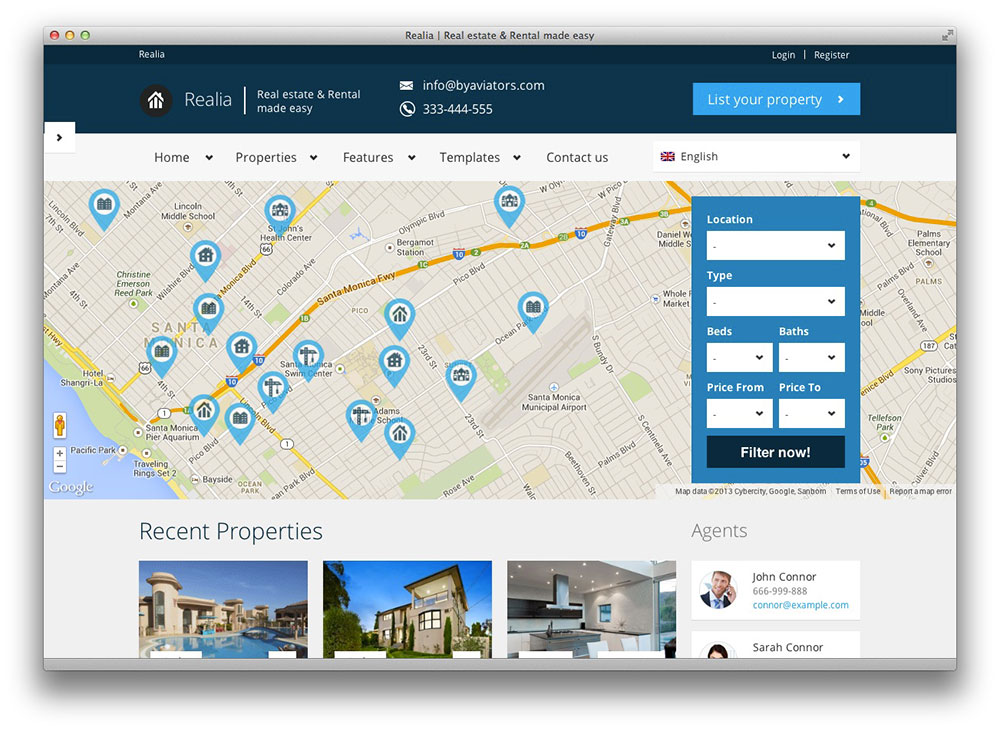The website homepage for Realia, as displayed in a web browser, prominently features the company name "Realia" in a dark blue banner at the top beneath the phrase "Real Estate and Rental Made Easy." Central to the banner is a black circle containing a minimalist stick-figure house icon adjacent to the text "Real Estate and Rental Made Easy." Contact details are provided as "info@byaviators.com" followed by a placeholder phone number "333-444-5555." Directly below, a light blue button labeled "List Your Property" invites users to take action. 

The navigation bar includes tabs for "Home," "Properties," "Features," "Templates," and "Contact Us." A drop-down menu for language selection defaults to "English."

A substantial map dominates the main section, marked with over a dozen blue location pins indicating various property listings. To the right of the map is a blue sidebar titled "Location," featuring multiple drop-down menus for refining searches by location, property type, bedrooms, bathrooms, and price ranges (from and to). At the bottom of this sidebar, a prominent rectangular black button reads "Filter Now," allowing users to apply their search criteria.